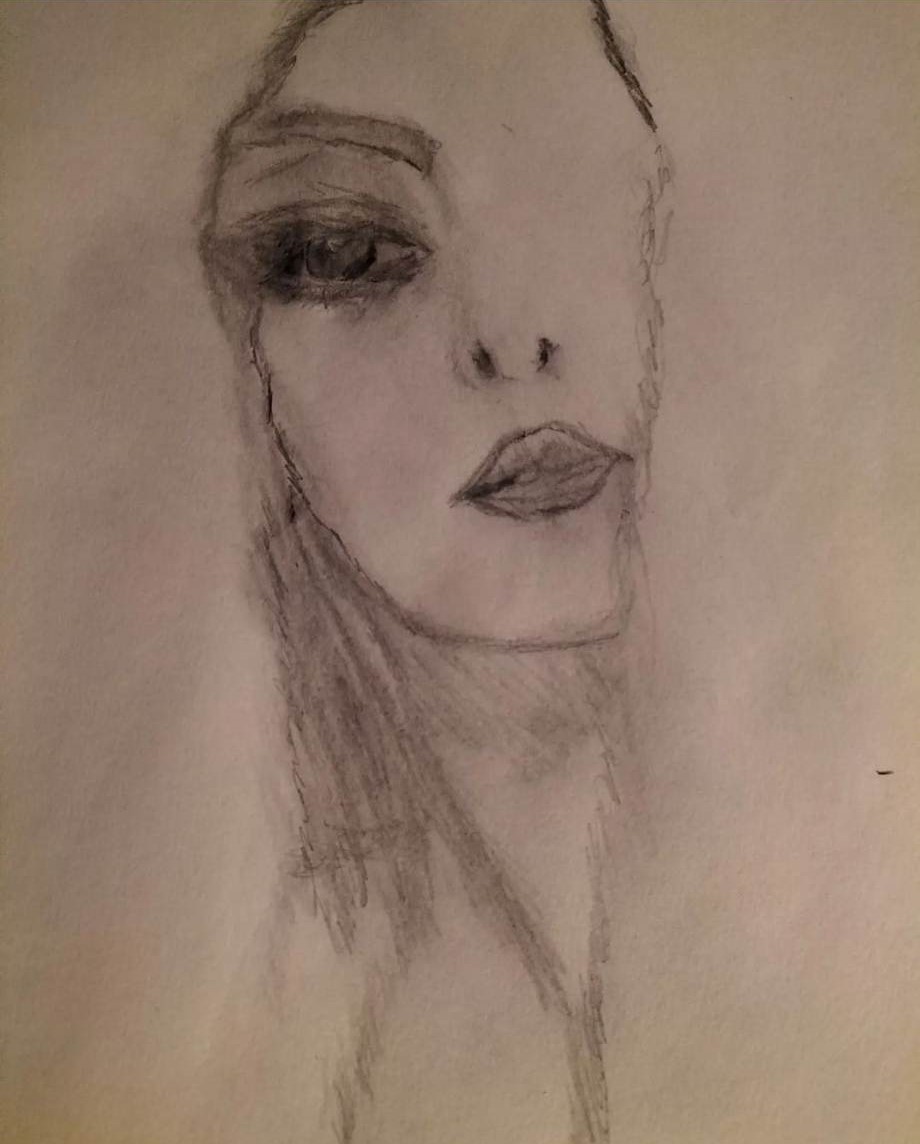This sketch, rendered on a piece of sketch paper, appears to be created with pencil, though it may also involve charcoal. Centralized towards the top middle of the paper, it showcases a partially-completed portrait of a girl's face. Delicate shading on the forehead transitions into lines that suggest hair, although the sides of the image remain blank, providing a stark contrast. The detailed left eye, complete with an eyebrow, prominently stands out alongside a meticulously drawn nose and mouth. The right eye remains unfinished. The girl has a distinct square chin with subtle shading underneath. She wears a V-neck top, and her lips are defined with lip liner, while her left eye features a deeply shaded, dark pupil.